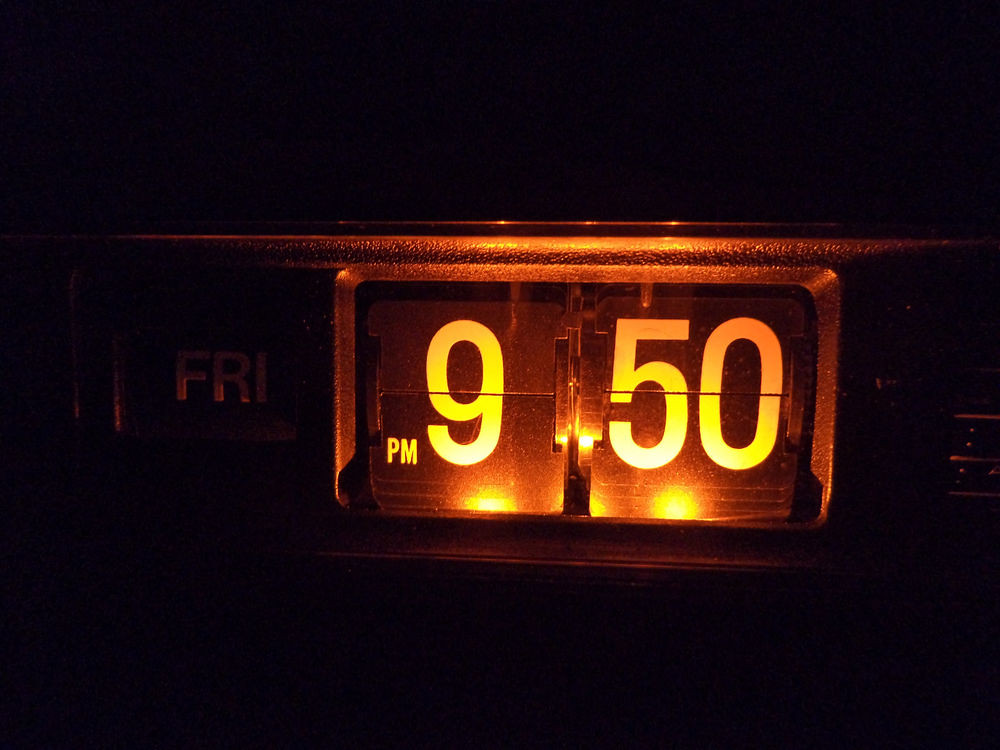This color photograph captures a striking image of an old-style, mechanical flip alarm clock, illuminated against an almost completely dark background. The glowing, sunset-orange to dark yellow light emanates from the base of the clock, highlighting the time display of "9:50 PM" in prominently bright numbers, and the day display "FRI" in smaller, adjacent lettering. The numbers and letters appear almost luminous against the dark setting. The clock's vintage design features black cards with white numbers that flip over, with visible dials and mechanical components around the display. The overall scene conveys a charming, nostalgic feel, emphasizing the sole illuminated elements in an otherwise black void.